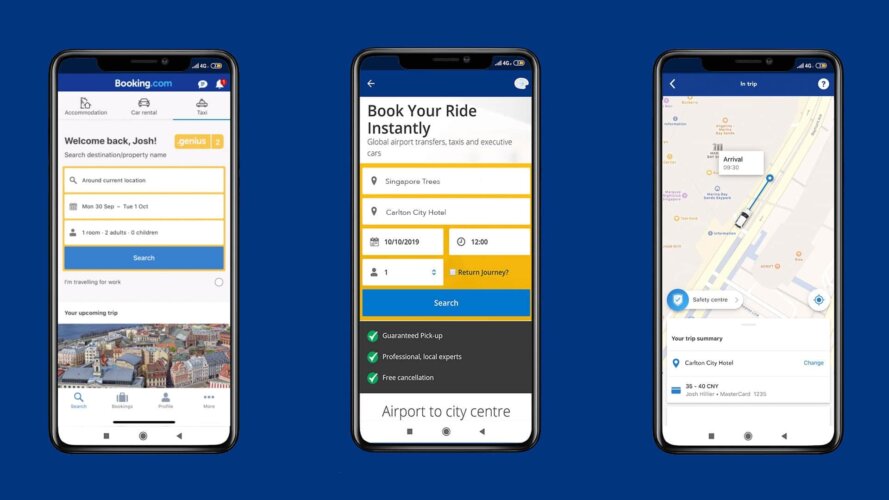The web page features a sophisticated and sleek dark blue background, prominently displaying three views of a cell phone, all highlighted in black. Each phone display illustrates different functionalities and information related to a trip or travel booking. 

On the rightmost phone screen, there is a detailed map showing a street view with a tiny car icon navigating the streets, indicating the current route of the trip. At the bottom, there's a trip summary detailing the journey to the Carleton City Hotel, accompanied by additional, albeit slightly illegible, details.

The middle phone screen features a dark blue banner at the top with the text in black reading, "Book Your Ride Instantly Global Airport Transfers Taxi and Executive Cars." Below this header, in bright yellow with white banners, it lists "Singapore Trees" and "Carleton City Hotel," specifying user destinations. Further down, it marks the date as 10-10-2019 and the time as 12 o'clock noon, with an icon of a person indicating one passenger. Below this is a blue search bar, under which a black section contains various elements including three checked green squares and the caption "Airport to City Center."

On the leftmost phone screen embedded in the layout provided by Booking.com, there is a section welcoming back a user named Josh. At the top, it features car rental options, a search icon for looking up information, and further details broken down into smaller boxes beneath. Toward the top of this display, a "Search" button is housed in a blue banner, while just underneath, a city view image appears with the heading "Your Upcoming Trip." At the bottom of the screen, several menu items are available for navigation.

This comprehensive layout caters to users seeking to book rides and plan their travels efficiently, with each phone screen providing distinct, yet interconnected pieces of information necessary for a seamless travel experience.